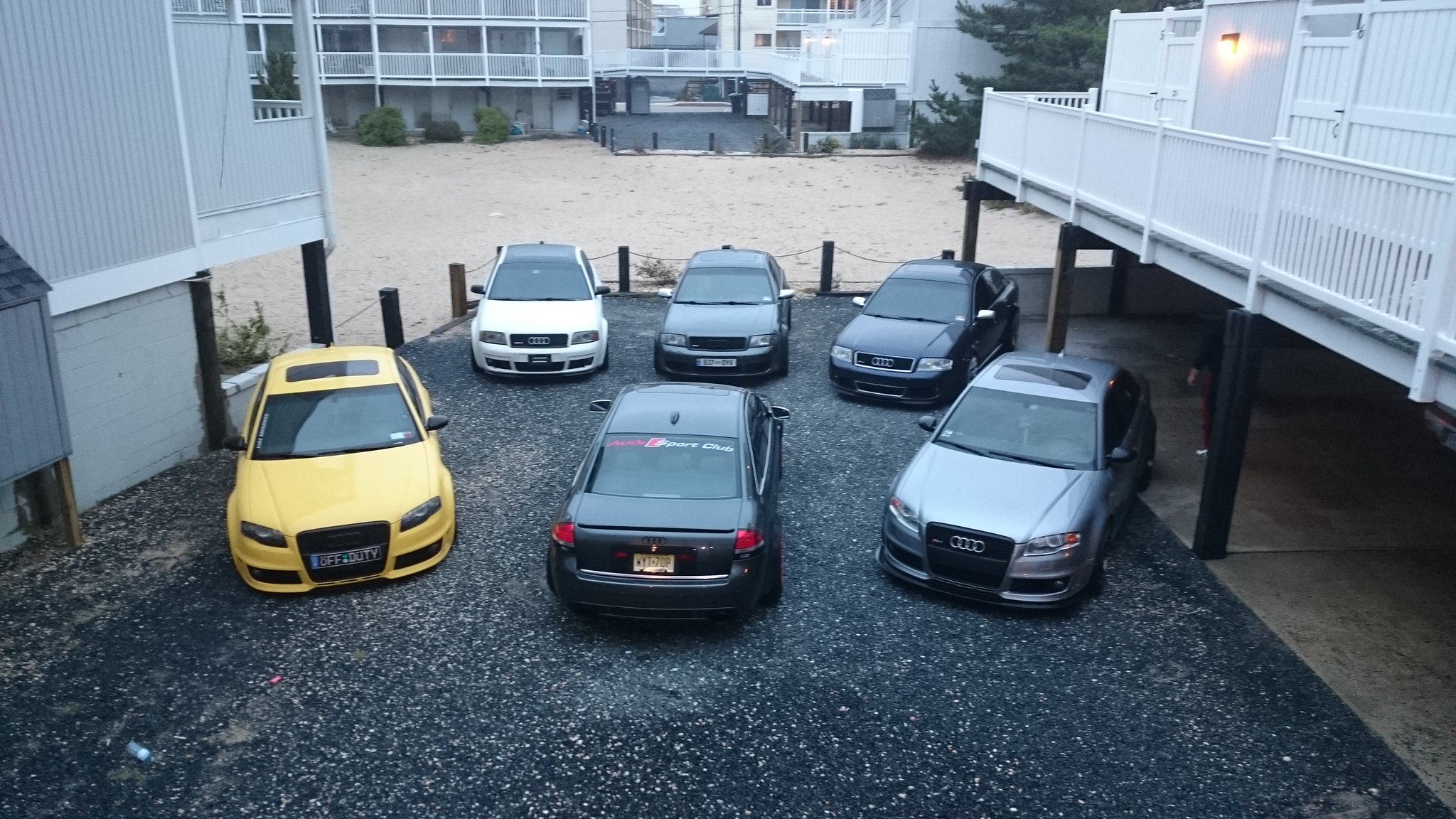The image appears to be taken from a second-story window, possibly from a pool area, looking down into a gravel-covered courtyard used as a parking lot between two white residential buildings. Both buildings are elevated on black stilts, creating an overhanging walkway for the one on the right side. Within the parking area are six cars arranged in two rows of three. In the closest row, there's a sporty yellow car with a European tag and a sunroof on the left, a black sedan facing away from the camera in the middle, and a silver Audi with a sunroof on the right. The back row features a white car on the left, a dark-colored car in the center—possibly black or green—and another black car on the right. Behind the parked cars, a white two-story building, resembling a mirror image of the foreground structures, is visible. The courtyard also includes telephone pole-like posts connected by ropes or chains, marking its perimeter, hinting at a possible river frontage location. The overall scene evokes a car enthusiast's interest, with the setting likely being a hotel or motel complex due to the architectural layout.